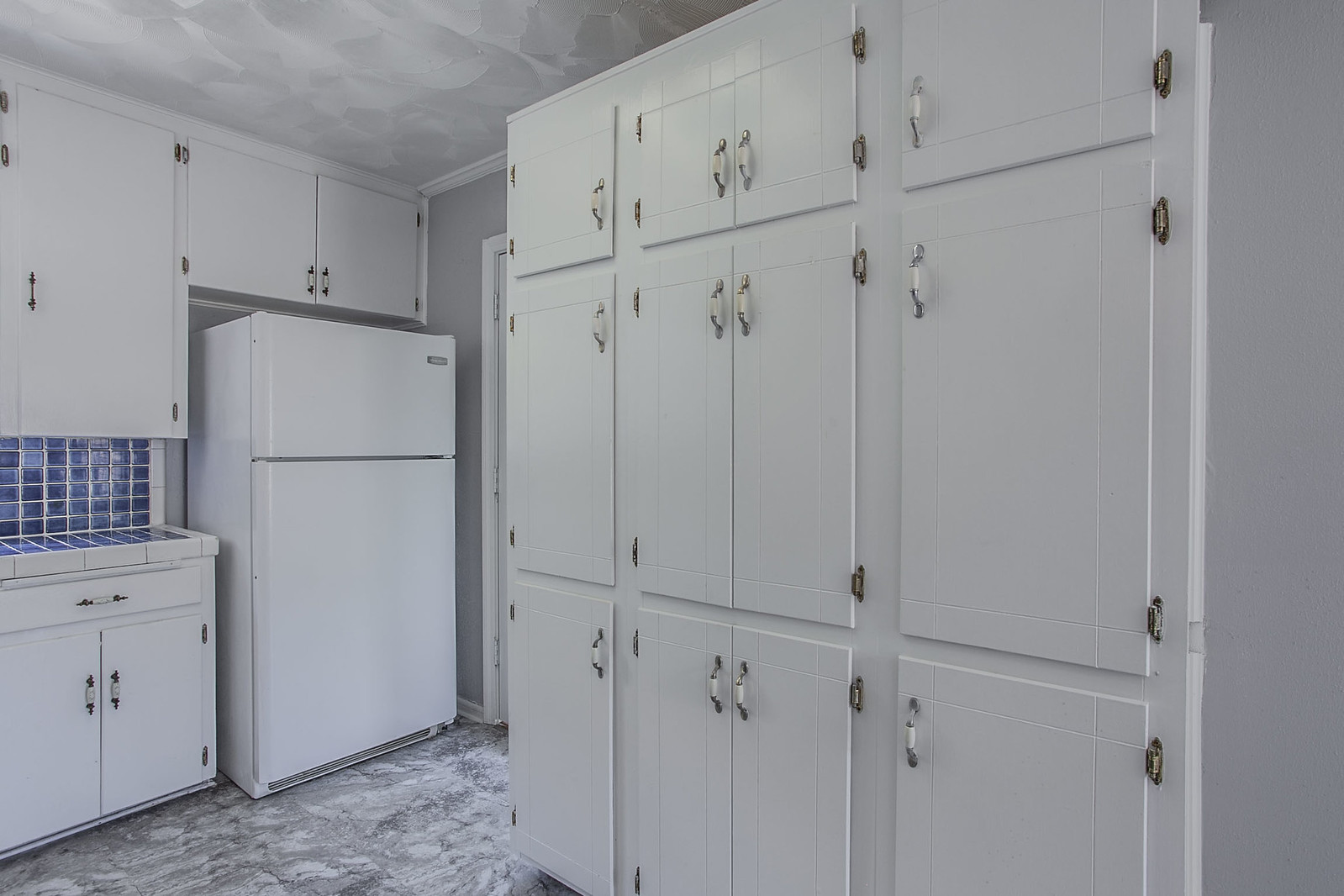This detailed photograph captures a stylish kitchen interior. The focal point is a white refrigerator with a smaller upper section for the freezer and a larger lower section for refrigeration. Surrounding the refrigerator are white cabinets, which feature elegant silver and white pulls. Specifically, there are smaller cabinets above and slightly larger ones to the left and right, including a set of pantry-like cabinets on the right side that are three rows tall and three columns wide. This cabinetry is uniform throughout, creating a seamless look. 

To the left of the refrigerator, there is a notable blue countertop and backsplash, featuring varying shades of blue that add a splash of color to the space. The flooring is a sophisticated faux marble pattern in white and gray resin, complementing the light gray or off-white walls. The ceiling is white with a distinctive wave or swirl pattern, adding a touch of texture to the room. The photograph effectively showcases the blend of white cabinetry, blue accents, and marbled flooring, giving an overall impression of a clean, modern, and cohesive kitchen design.